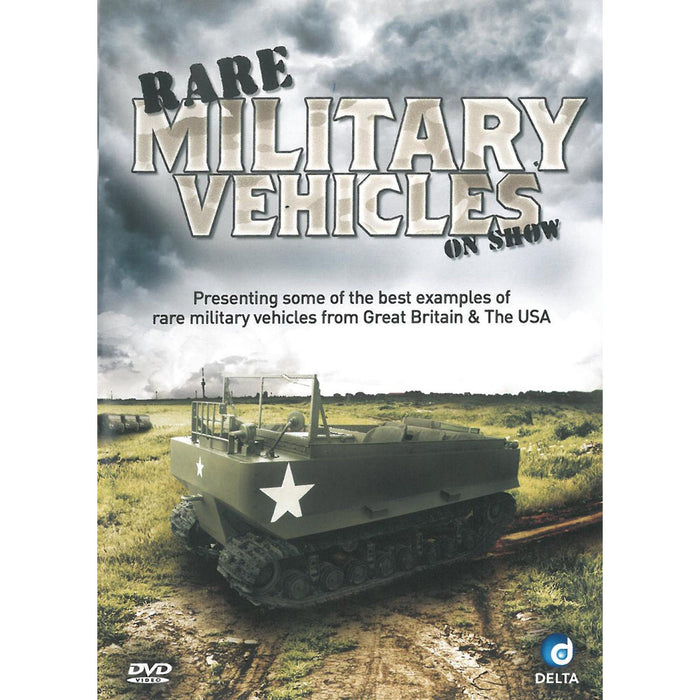The image is a DVD cover for a documentary titled "Rare Military Vehicles on Show." The title appears at the top, with "Rare" written in black text at a slant, and "On Show" positioned below the 'S' in "Vehicles," also in a slanted black font. The words "Military Vehicles" are prominently displayed in large, semi-translucent white text, blending slightly with the cloudy sky background. Below the title, in smaller text, is the subtitle: "Presenting some of the best examples of rare military vehicles from Great Britain and the USA." The centerpiece of the image features a green military vehicle resembling a tank, adorned with white stars, and designed with treaded wheels for traversing diverse terrains like snow or sand. This vehicle lacks a prominent cannon, suggesting it might be a transport vehicle rather than a combat tank. The background showcases a marshy, wet landscape with dark clouds gathering in the sky, giving the scene a dramatic effect. At the bottom left corner, the cover identifies the format as "DVD video" in white text, and the bottom right corner features the Delta company logo.